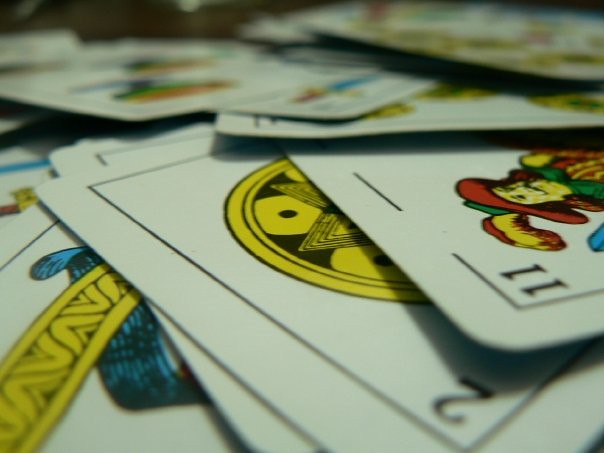This detailed image captures an intimate close-up of what appears to be a selection of gaming cards, intricately laid out and somewhat overlapping each other. The composition of the photo brings the viewer’s focus to a few central areas that are sharply in focus, highlighting the vibrant details of the cards. Dominating the scene on the right is a card marked with the number eleven, featuring a flamboyant character. This character is adorned in a wide-brimmed red hat, complete with a feather, evoking the image of a jester. His outfit combines vivid hues of red, green, and yellow; he sports a red suit with striking yellow sleeves and a green tie. Adjacent to this card is another featuring the number two. Although partially obscured by the eleven card, it prominently displays a yellow circle at its core, filled with intricate black designs. Within this circle, one can discern a star motif providing a stark contrast. The background reveals more cards, descending in a blur that conveys depth and motion, emphasizing the card pile's intricate and dynamic nature.